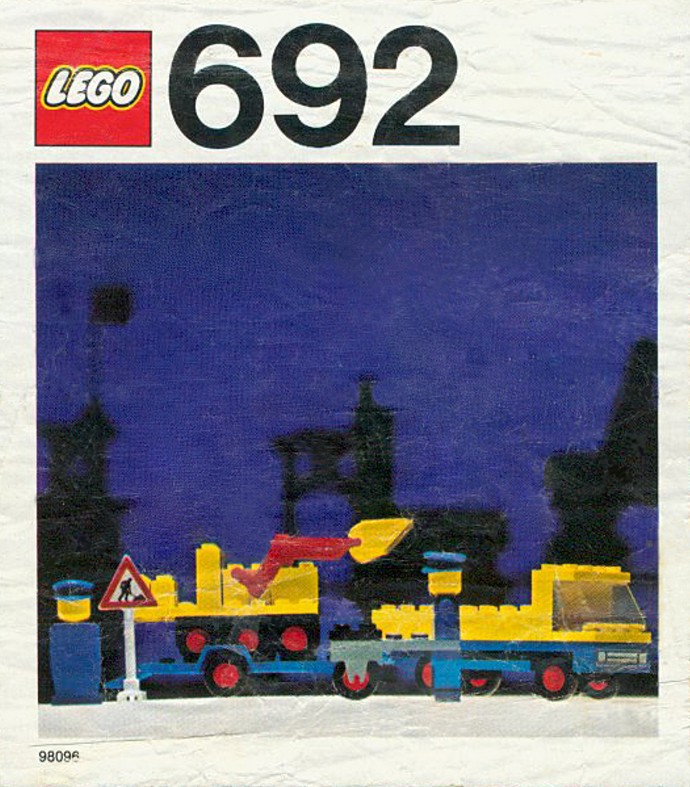This is a square, time-worn image of Lego Set 692, seemingly scanned from a wrinkled paper print. The traditional Lego logo, a red square with "Lego" in balloon-like white letters, prominently occupies the top left corner. Beside it, the number "692" is displayed in large black print. Below the logo and set number, within a large square area of dark blue background, the main focus is a detailed Lego construction scene.

The scene showcases a yellow construction truck hitched to an excavator, both made entirely of Lego bricks. The excavator appears to be in the act of dumping something into the truck. Two Lego figures, possibly representing police officers or construction workers, stand nearby, watching the operation. These figures are dressed in uniforms that align with their roles in the miniature construction setting. Adding to the sense of activity, a triangular Lego hazard sign depicting workers lends authenticity to the scene. Overall, this nostalgic image encapsulates the playful and intricate world of Lego building, bringing to life a construction yard bustling with activity.